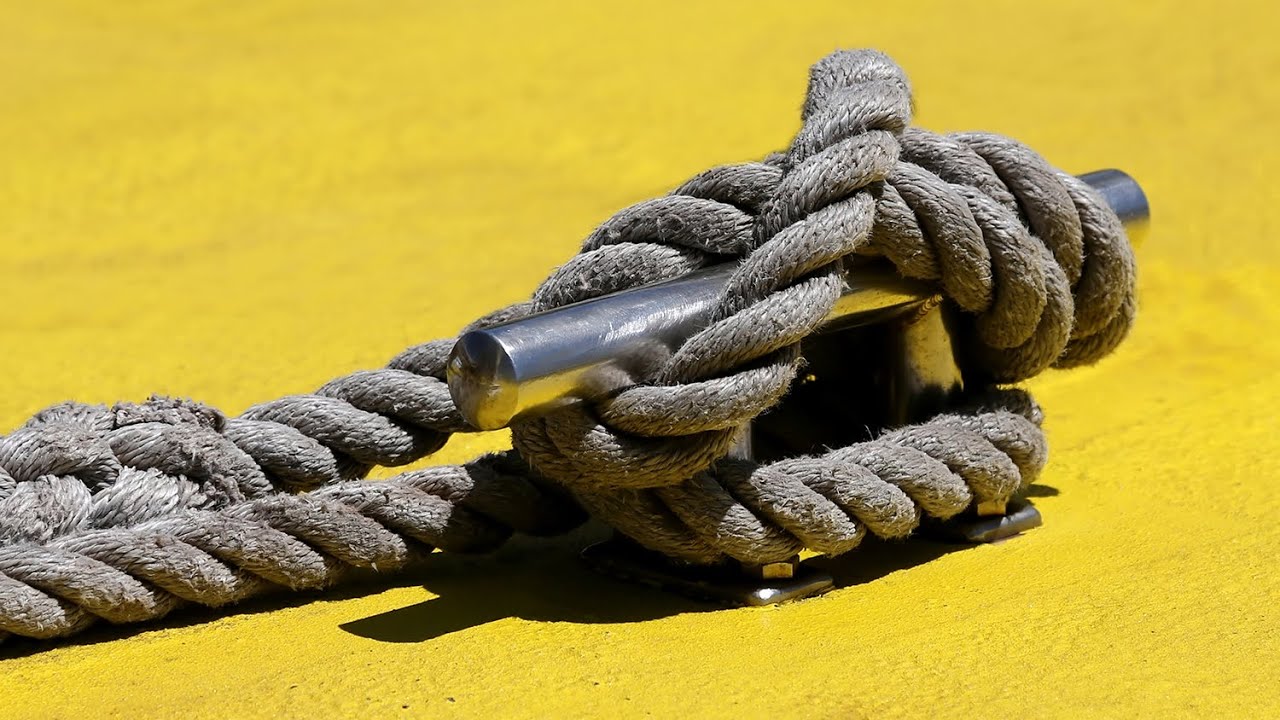This photo features a close-up view of a thick, frayed, dark gray nautical rope securely tied around a sturdy, shiny silver cleat. The cleat, which is anchored with several nuts barely visible beneath the rope, is affixed to a flat yellow surface that appears to be painted, as evidenced by small worn spots. The yellow surface, likely part of a dock, provides a cement-like texture in the background. On this bright sunny day, the rope and cleat cast clear shadows on the surface. The rope itself, approximately an inch and a half to two inches in diameter, extends out of the frame on the left side, leaving its attachment point to the boat or dock unseen. The overall impression is one of durability and strength, suggesting the boat is securely moored.